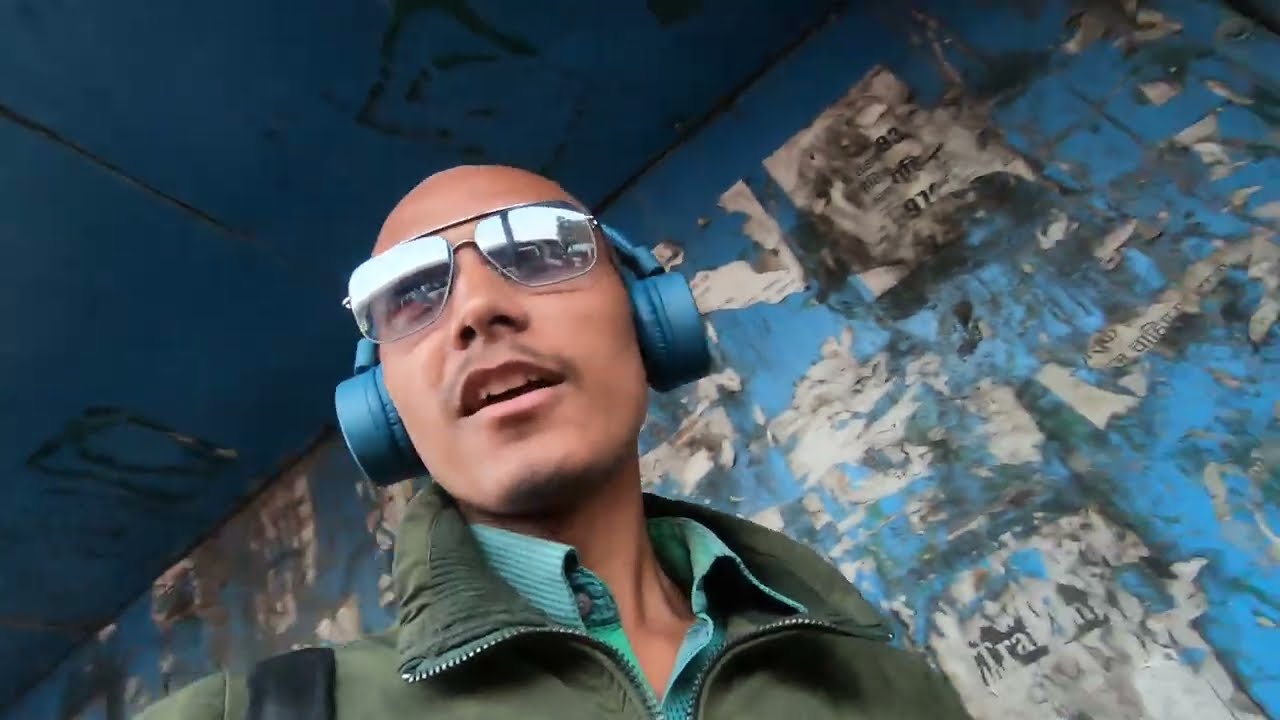The image features a man with an olive complexion or tan skin, possibly Latino, positioned centrally. He is slender with a completely shaved head and has a faint mustache and a slight goatee. The man wears tinted aviator-style glasses and blue over-the-ear wireless headphones with padded ears. His attire includes a green zip-up jacket over a turquoise button-down shirt with the top button undone. A black strap is visible on his left shoulder. The background consists of a blue wall and ceiling, appearing weathered and dirty with numerous torn and scraped-off posters or stickers, suggesting a gritty urban environment. The photograph is taken from a slightly low angle, making it seem as though the camera is positioned just below his face, capturing him from the shoulders up as he appears to be mid-sentence.